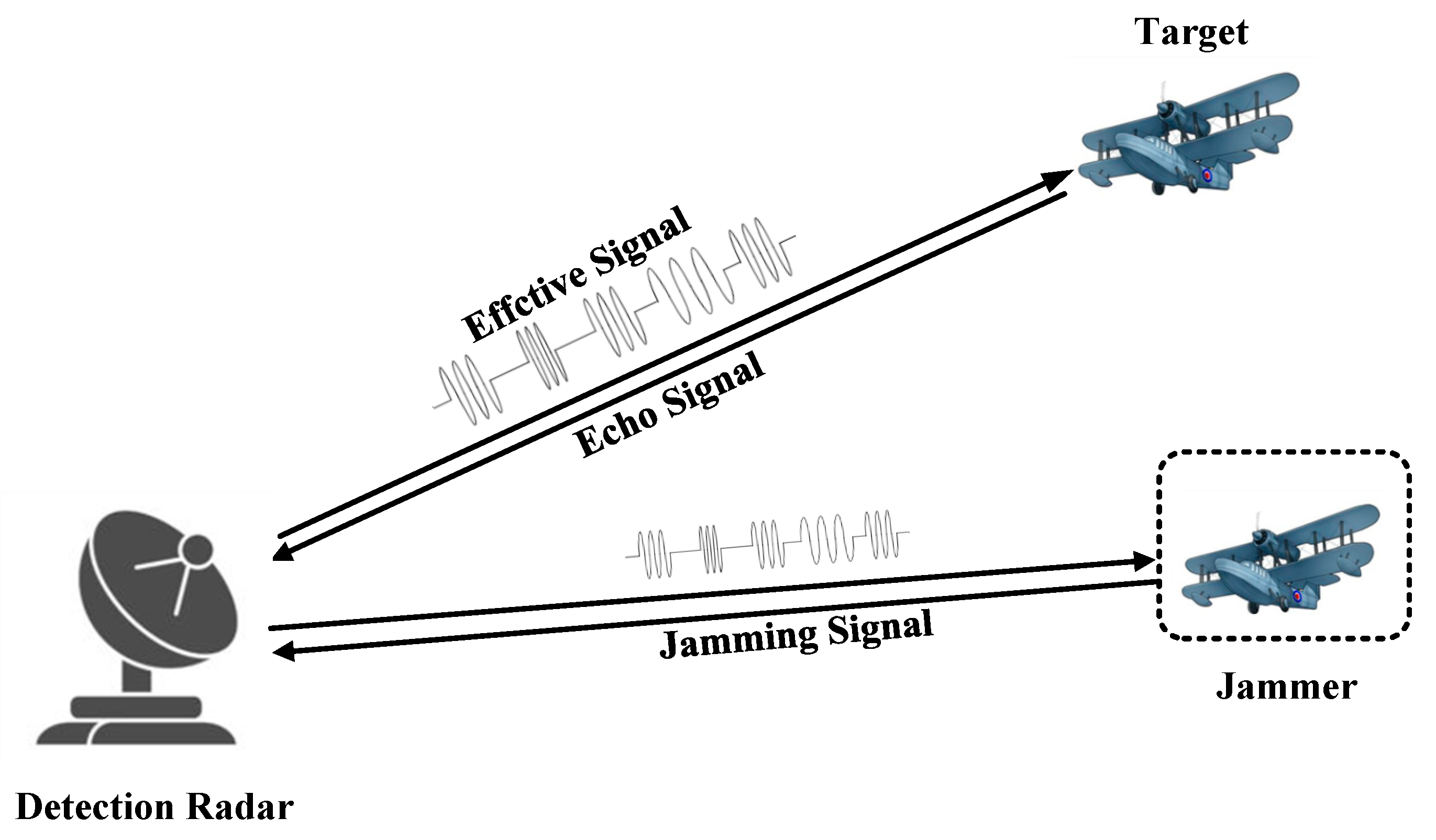This detailed illustration depicts the functioning of detection radar and the concept of jamming. On the left side, a basic drawing of a satellite dish labeled "Detection Radar" points to the right. Above the dish, arrows labeled "Effective Signal" and "Echo Signal" extend to an old biplane, which is situated in the upper right-hand corner and labeled "Target." The signals are represented by swirly lines, symbolizing radar waves. Below this, another set of arrows, labeled "Jamming Signal," point towards a second biplane, identical in appearance but surrounded by dashed lines and labeled "Jammer." This instructional illustration utilizes a color scheme of black, white, gray, and blue, with a hint of red on the decal of the planes. The entire image is designed to demonstrate how radar signals detect targets and how those signals can be disrupted by jamming.